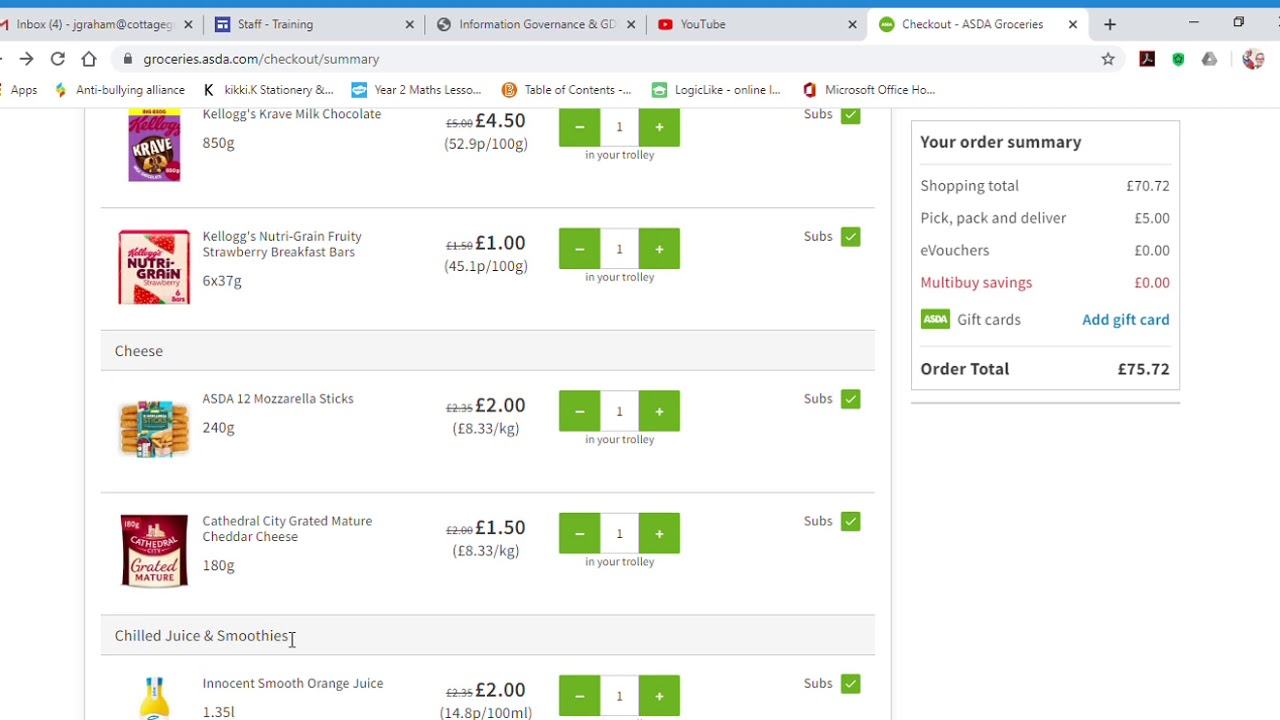The image captures a detailed screenshot of the webpage groceries.asda.com, showcasing an online grocery shopping experience. The user has an array of different food products in their virtual shopping trolley, with their cart organized in various sections.

At the top of the list, Kellogg's Krave Milk Chocolate cereal is displayed, indicating that there is one unit of this product in the trolley. Similarly, the shopper has added one Kellogg's Nutri-Grain Fruity Strawberry Breakfast Bar. A green checkmark is present in the substitutions box, suggesting that the shopper agrees to receive similar items if their selected products are unavailable.

The cheese section includes ASDA’s own brand of 12 Mozzarella Sticks and one packet of Cathedral City Grated Mature Cheddar Cheese. Additionally, the beverages section features one bottle of Innocent Smooth Orange Juice, a likely favorite brand of the user.

The overall summary of their order comes to approximately £70, with an additional £5 fee for picking, packing, and delivery services, rounding the total to £75.72.

The screenshot also reveals an array of other open browser tabs, including YouTube, a staff training page, an information and governance tab, and an email client, hinting at the user's multitasking routine.